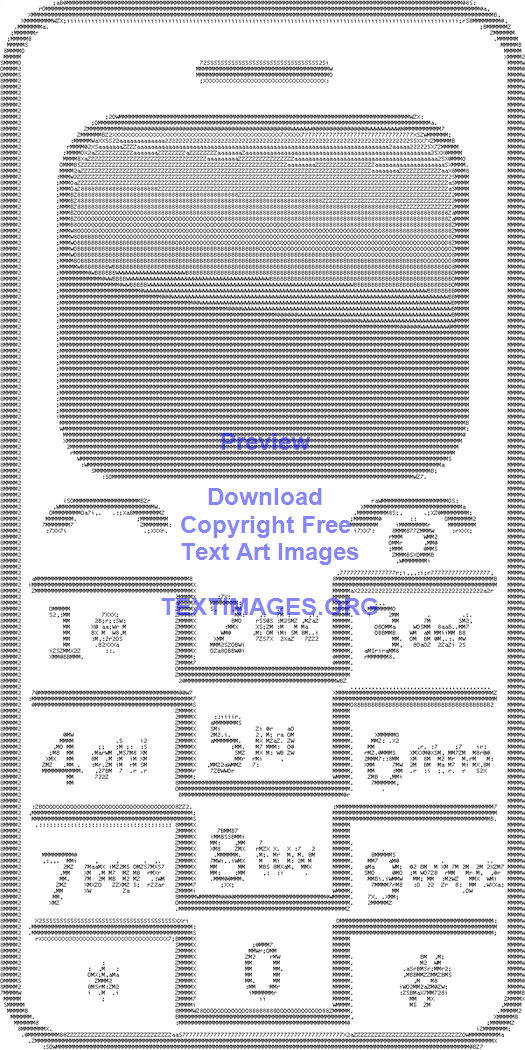This detailed image depicts an old-style cell phone created entirely from text characters, numbers, and letters, showcasing a form of text art. The cell phone, rendered in black and white, features a traditional keypad with numbers 1 through 9, alongside the * and # symbols. The characters 2, 5, and 8 also have their associated letters (ABC, DEF, etc.) next to them. The shading and detailing with these text characters result in a highly realistic depiction of the phone. Overlaid on the image is a blue watermark that reads, "Preview Download Copyright Free Text Art Images textimages.org." This watermark suggests the source of the text art and extends across the image, which covers the entire frame. The unique use of text to outline the handset, the screen, and the keys illustrates the artistic technique of forming images through textual characters, enhancing the vintage technological theme of the artwork.